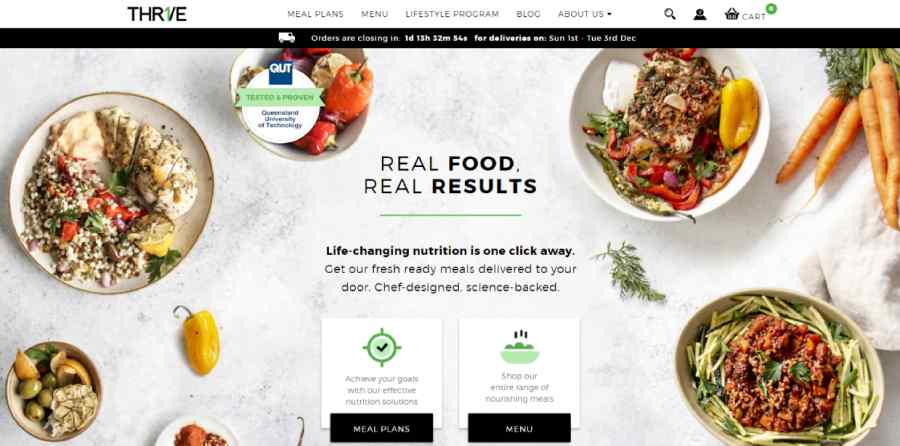This screenshot showcases a food delivery website named "Thrive." At the top, the website's logo "Thrive" is prominently displayed, with a distinctive green section on the first part of the "V". The navigation menu features multiple headings: 'Meal Plans', 'Menu', 'Lifestyle Program', 'Blog', and 'About Us,' with the latter opening to a dropdown menu. Along this same line, you can find icons for search, user ID, and a shopping cart.

Just below the menu, a black banner dominates the screen, featuring a central white icon and the urgent message: "Orders are closing in one day, 13 hours, 32 minutes, and 54 seconds for deliveries on Sunday, the 1st, Tuesday, 3rd, December."

The main body of the screenshot displays appetizing food images, drawing attention immediately to a large plate on the left. This rustic beige plate contains a well-arranged meal of chicken, rice, and vegetables, complemented by a yellow pepper resting on the counter. Nearby, a bowl filled with red peppers adds a splash of vibrant color to the scene.

At the center, a bold message reads: "Real food, real results. Life-changing nutrition is one click away. Get our fresh, ready meals delivered to your door, chef-designed, science-backed." Below this statement, two squares are followed by two prominent black buttons labeled 'Meal Plans' and 'Menu'.